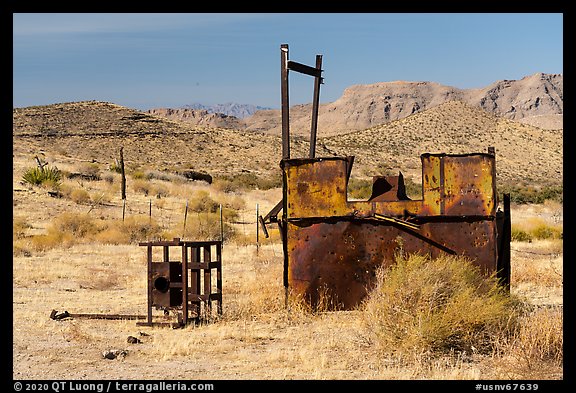The image is a framed photograph with a black border. In the bottom left corner, in white text, it reads "Copyright 2020 QT Luong / Terragalleria.com," and in the lower right corner, it says "US NFS 67639" in small text. The scene depicted is a desert landscape dominated by dry, sandy, and beige mountains in the background, with minimal vegetation. In the middle ground, some slight vegetation and flat-topped hills are visible under a stretch of blue sky occupying the top third of the image. The foreground is populated with tumbleweeds and dried grass clumps. A prominent feature in the scene is a rusted, rectangular piece of metal machinery, likely old mining equipment, marked by yellow and brown rust. Adjacent to this structure is another stand-like equipment, possibly a heater, also rusted. Scattered around the scene are rusted sheets of metal and what appears to be a darker, rusted metal table. The overall setting evokes a stark and abandoned desert atmosphere.